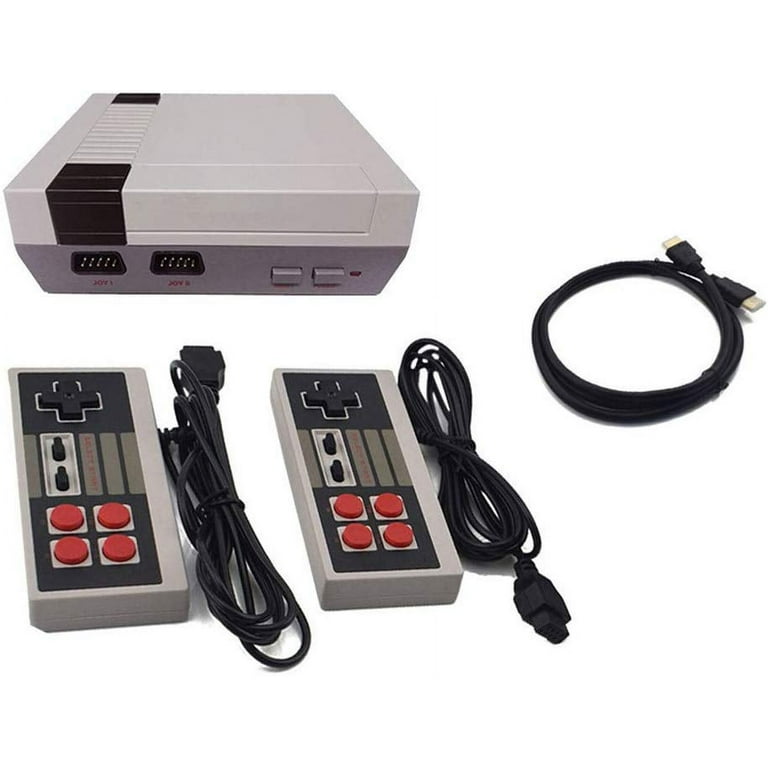This is a detailed color photograph in landscape orientation, featuring an older model Nintendo mini gaming console set against a white background, creating an impressionistic floating effect. The light gray and dark gray rectangular console sits at the top left, equipped with multiple plugs for electrical connections. The console includes power switches and slots labeled "Joy 1" and "Joy 2," indicating ports for the controllers. The cartridge slot on the console has a pull-up design for game insertion.

Below the console, two corded handheld controllers are positioned vertically. Each controller, with its coiled black power cord neatly bundled beside it, showcases four red buttons and a black D-pad with two small black levers at its center. A separate coiled connecting cord with visible ends lies to the right of these items, further emphasizing the retro design of the system.

The detailed photographic representationalism realism style captures the essence of this classic gaming system, highlighting its nostalgic features and design elements.